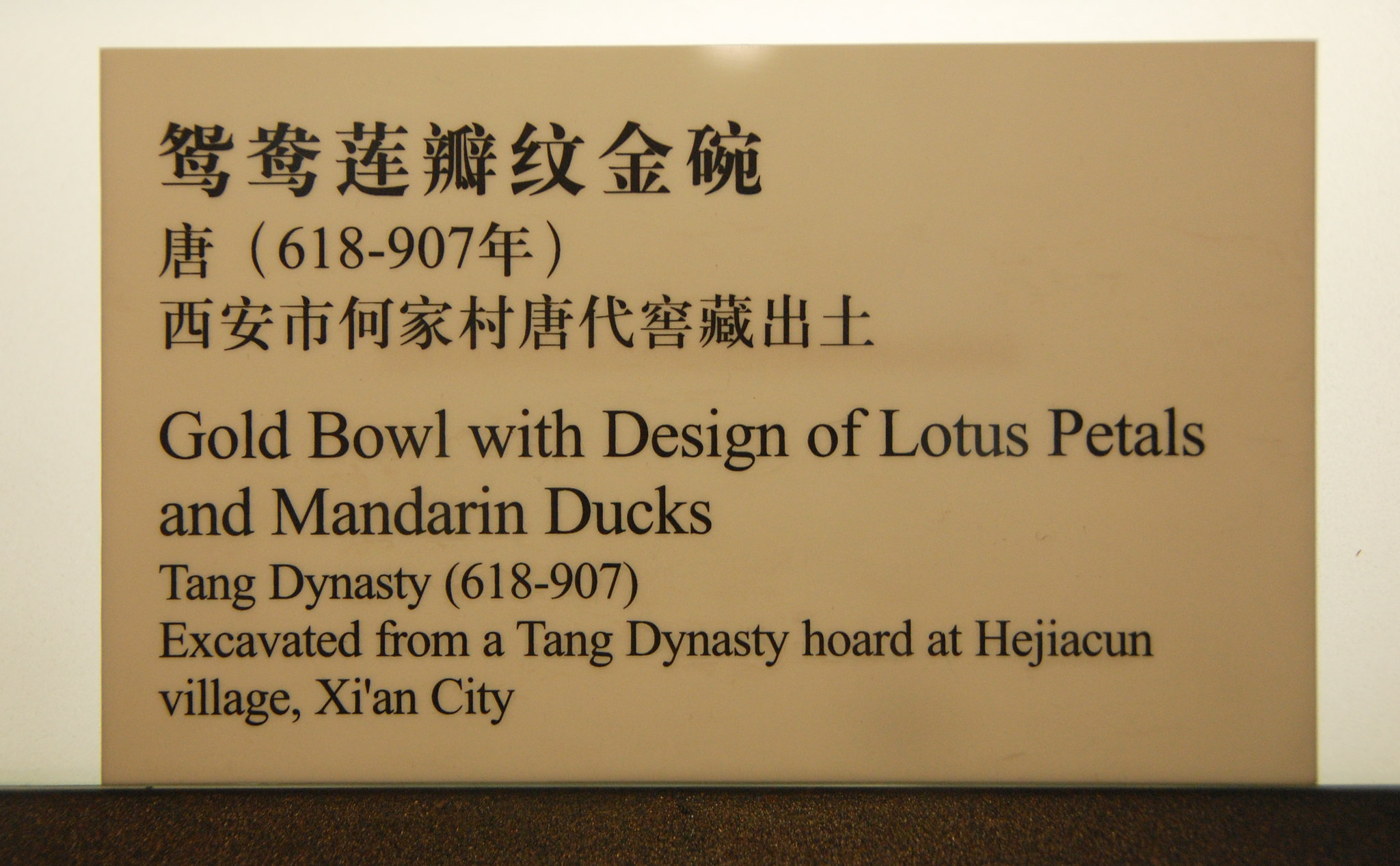This image depicts a rectangular sign with a medium brown background layered over a beige background, placed on a table. The sign features Chinese characters on the first line, flush with the left-hand side. The second line contains a Chinese character followed by the numbers "618-907" in parentheses, and then another Chinese character. Below these, another line of Chinese characters is present. 

Beneath the Chinese text, in large English print, the sign reads: "Gold Bowl with Design of Lotus Petals and Mandarin Ducks, Tang Dynasty." Following that, in parentheses, it shows the years "618-907". The sign states that the item was excavated from a Tang Dynasty hoard at Heijia Kun Village, Xinyi City. The text is predominantly black, and the sign has a white frame around the top, left, and right sides, while the bottom part contains a darker brown with black and white flecks.